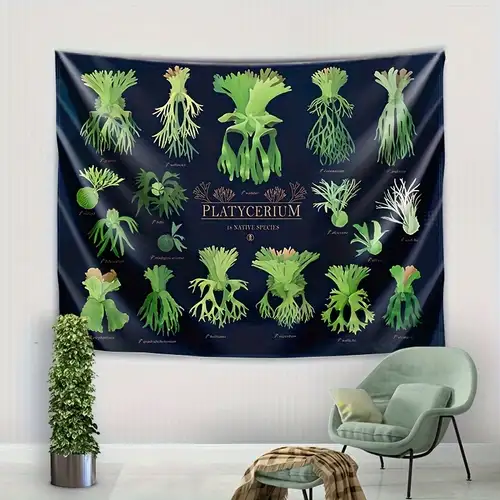The image features a gray wall adorned with a vibrant tapestry showcasing various green plants. The banner displays five distinct plants at the top, the central one being the largest. Below these, four bulbous plants with green leaves form a cluster on the left, while three similar plants are arranged vertically on the right. Gold lettering in the center reads "PLATYCERIUM," signifying a native species. The bottom row of the tapestry illustrates six plants of varying sizes, with their roots visible. In the bottom left corner, a silver pot contains a tall, slender plant. To the lower right, a grayish-blue plastic chair with matching cushions and a small white pillow is positioned near a stool draped with a brown and light-brown cover.